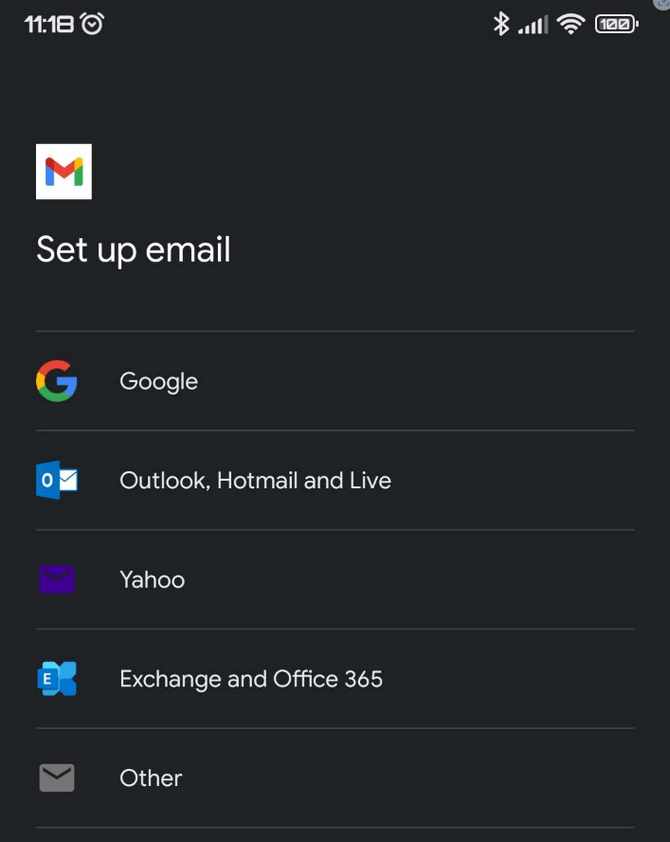A smartphone screen displays an interface with a black background. The time "11:18" is shown at the top, accompanied by icons for an alarm clock, Bluetooth, a strong cellular signal represented by four out of five bars, full Wi-Fi connectivity, and a fully charged battery at 100%.

Below these icons is a white square featuring a stylized "M" composed of colorful segments in yellow, orange, red, and blue hues. Underneath this square, white text reads "Set up email." A light gray line extends almost the full width of the screen below this text, stopping just short of the edges.

Further down, the interface includes the Google logo, with a capital "G" next to the word "Google." Below another gray line, there is an envelope icon followed by the text "Outlook, Hotmail, and Live." Additional gray lines segment the screen into sections with different icons and text. A purple "Y" denotes Yahoo, followed by a blue icon indicating "Exchange and Office 365." Finally, a gray envelope icon is labeled "Other."